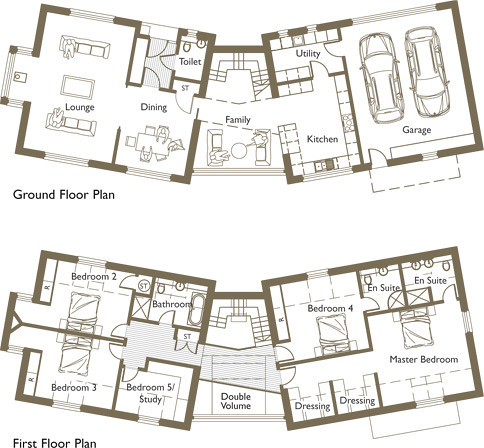The image features two architectural blueprints arrayed vertically. 

The top blueprint, labeled "Ground Floor Plan," consists of two rectangles angled toward each other at their top edges, connected by two lines—one shorter on top and one longer on the bottom. Inside, several rooms are clearly outlined and labeled. On the left side, there's a doorway leading into a rectangle marked "Lounge," furnished with two couches. Adjacent to the lounge, on the right, is a smaller square labeled "Dining," featuring a dining table. Opposite the dining area is a space labeled "Toilet." The central section of the blueprint is designated as "Family." Moving right, there's a larger rectangle split into two sections: the "Kitchen" and a smaller "Utility" area. The far right edge of the blueprint houses the "Garage," showcasing two cars parked in opposite directions.

The bottom blueprint is labeled "First Floor Plan." On the left side, it is segmented into "Bedroom Three" at the bottom and "Bedroom Two" at the top. Adjacent to these, two smaller rooms are labeled "Bathroom" (at the top) and "Bedroom Five/Study." The middle section bears the label "Double Volume." To the right of this, a square denotes "Bedroom Four," beneath which are two smaller rooms each labeled "Dressing." On the far right, a square space is labeled "Master Bedroom," topped by two smaller squares both marked "En Suite."

Together, these detailed floor plans present a comprehensive layout of the ground and first floors of a residence, highlighting the spatial arrangement and specific designations of each room.